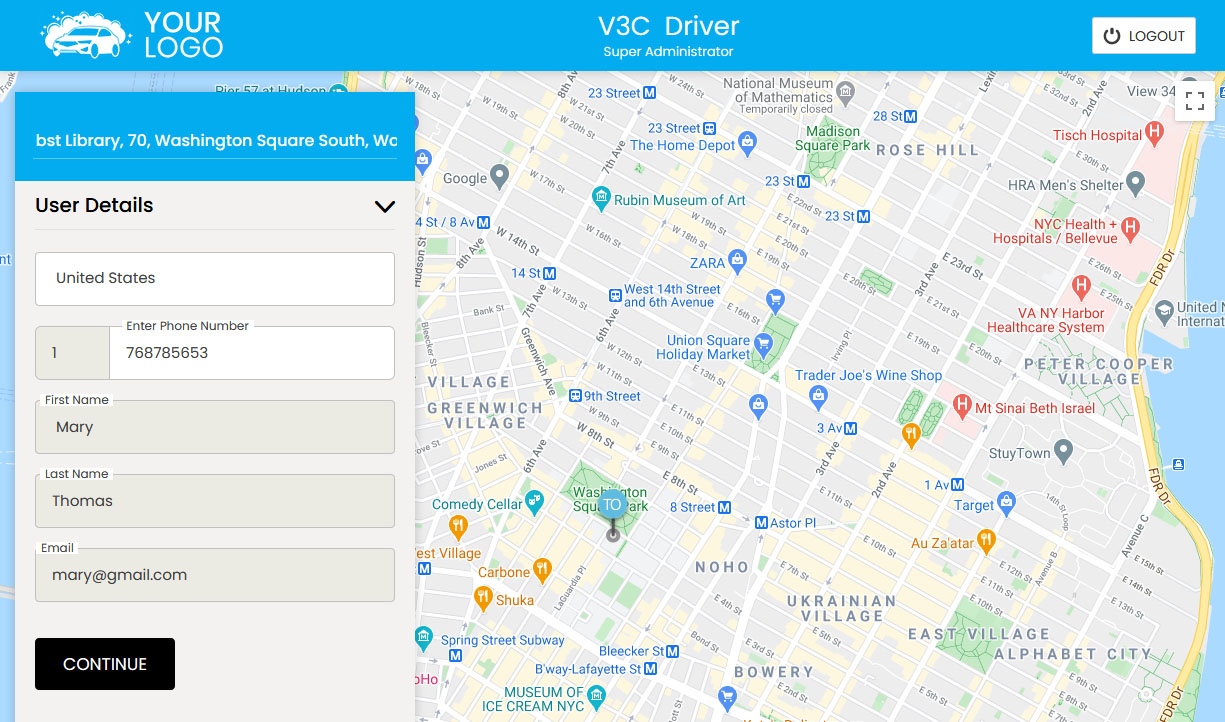In this image, the majority of the frame is dominated by a large map. The map appears to be a standard street map, with various locations and streets highlighted. To the right of the map, there is a small body of water. Specific landmarks and locations are indicated in different colors: some locations, such as NYC Health + Hospitals/Bellevue and B-A-N-Y Harbor Healthcare System, are highlighted in orange text. Other locations, including Union Square Holiday Market, Trader Joe's Wine Shop, 23rd Street, and The Home Depot, are marked in blue text.

At the top of the map, there is a blue bar that features a small car graphic on the left side. Next to this graphic, "Your Logo" is written in white text. The middle section of the bar reads "V3C Driver" and directly below it, "Super Administrator" is noted. On the right side of the blue bar, there is a logout button.

On the left side of the image, there is a box labeled "User Details." Inside this box, user-specific information is displayed. The selected country is the United States, and the user has entered a phone number, the name "Mary Thomas," and an email address "mary@gmail.com." Beneath these details, there is a black button with white text that says "Continue."